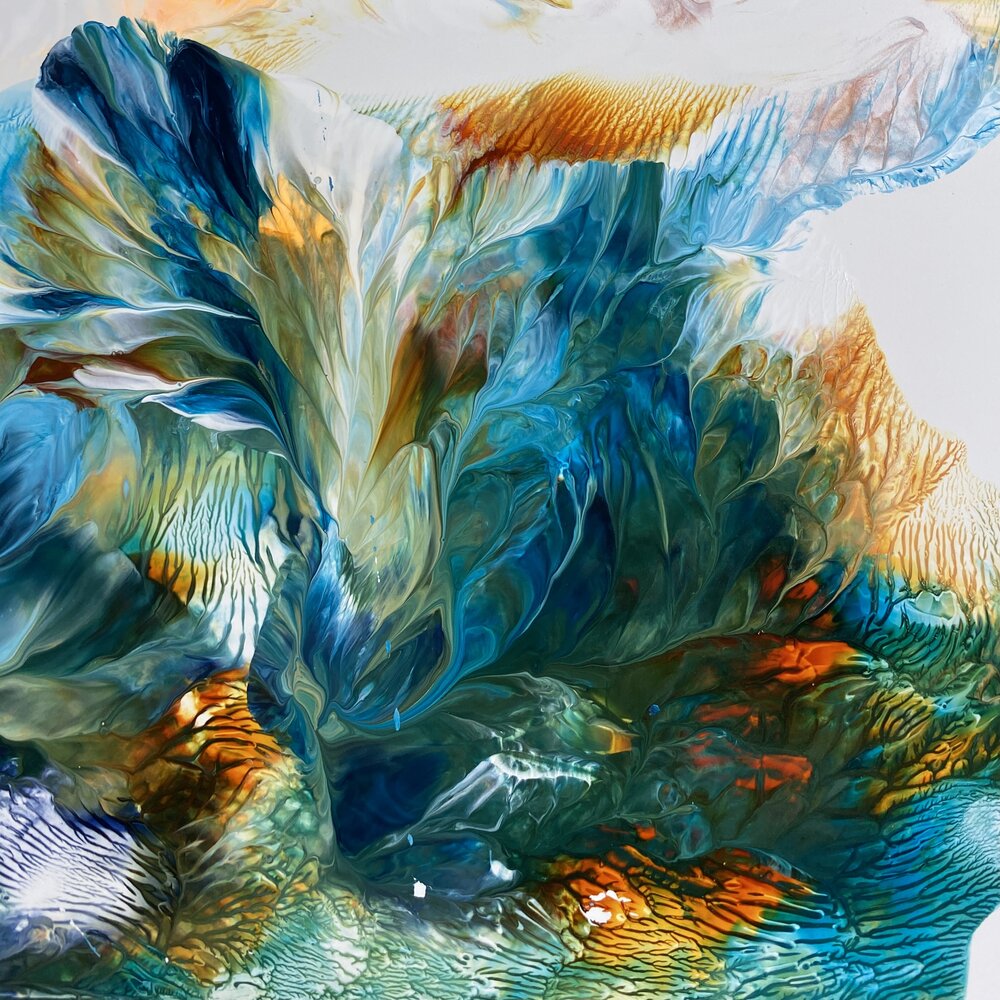The painting is an abstract watercolor artwork created using the marbling technique on a wet canvas, allowing the colors to bleed and swirl into one another. This creates an ethereal, fluid composition with shades of turquoise, light blue, dark blue, teal, white, rusty orange, pale peachy orange, gold, and brown. The colors intermingle and streak together, forming a visually striking pattern that resembles spiraling ocean waves with leaping fish, or perhaps multicolored flames. The intricate swirls and towers of color evoke a sense of movement and dynamism, with the bottom portion resembling water ripples and the top becoming more streaked as the colors merge and spiral upward. The pure white background accentuates the vivid, swirling colors of the painting.